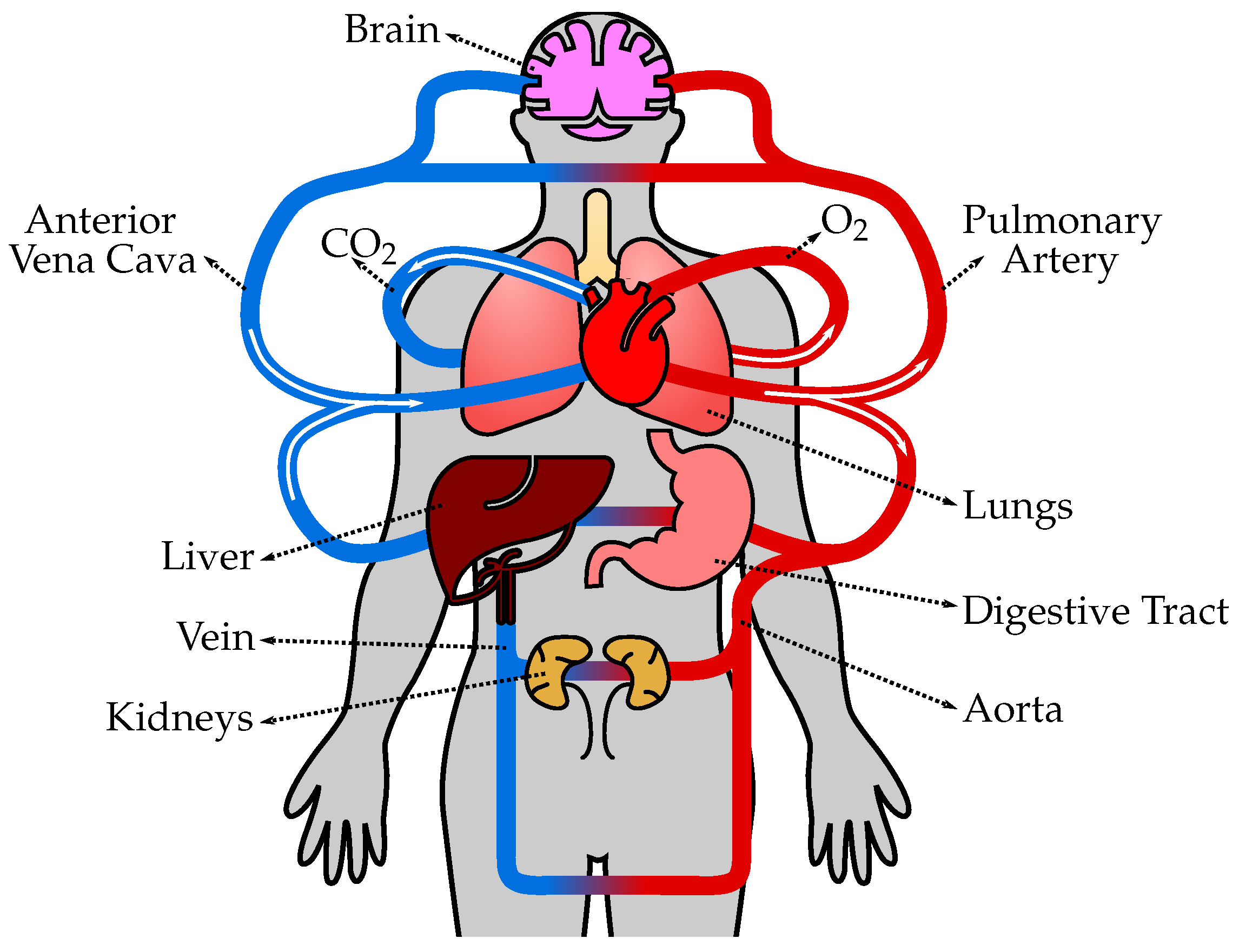This is an animated drawing of the human body, focusing on the anatomical layout from the hips up, depicted in gray. The diagram is labeled with key anatomical parts: the brain at the top, the anterior vena cava, the pulmonary artery, the aorta, the lungs, the liver, veins, the kidneys, and the digestive tract. Each organ is illustrated within the body, with blue and red lines highlighting the pathways of blood flow—blue lines indicating the flow of blood containing carbon dioxide (CO2) and red lines indicating blood carrying oxygen (O2). The labels provide additional details such as the interior vena cava for the blue pathway and the pulmonary artery for one of the significant red pathways. Overall, it presents a simplified but comprehensive overview of human anatomy and blood circulation, suitable for a basic medical textbook.